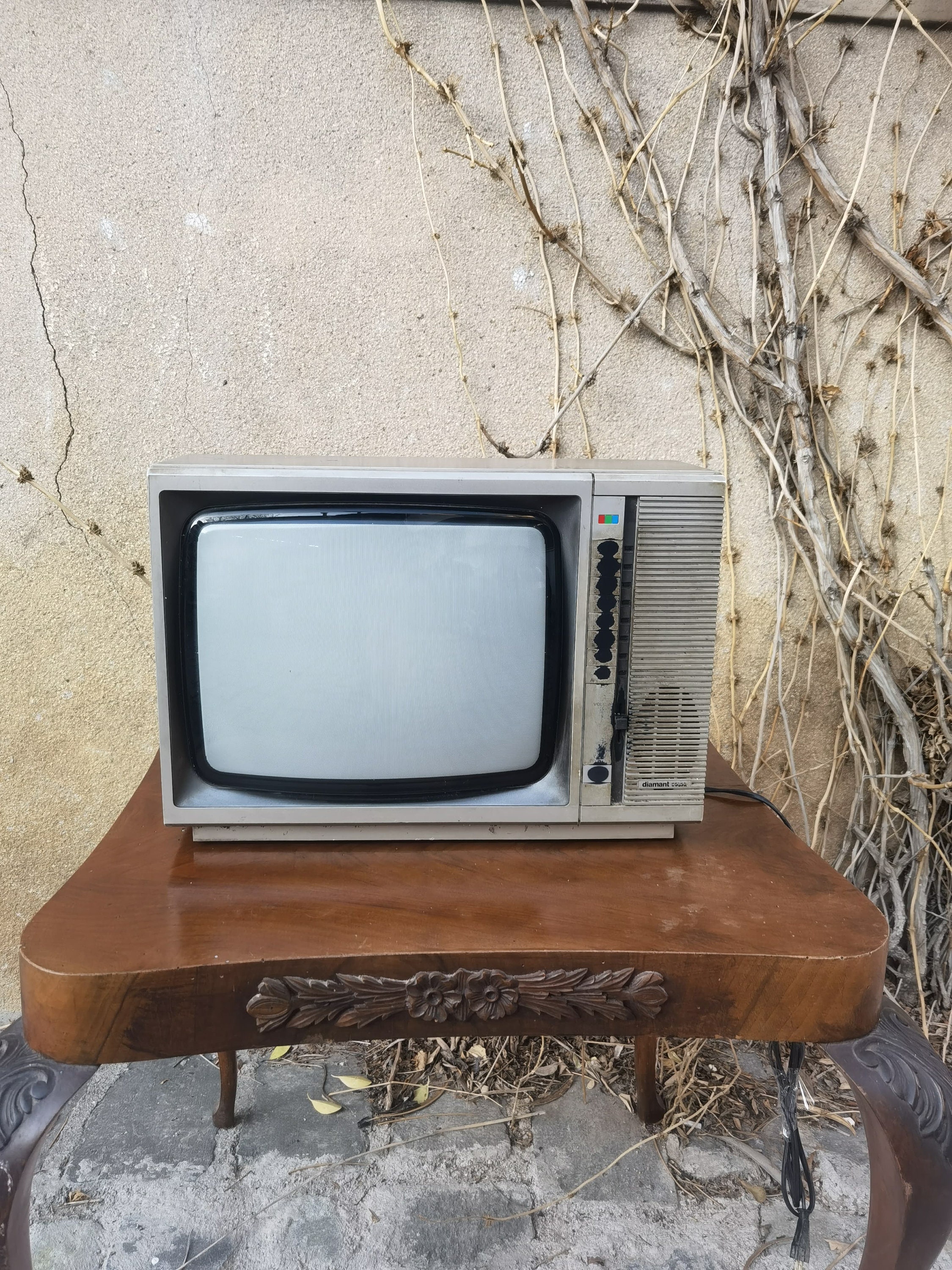In this image, we see an antique box television in a gray plastic casing, with a small, light gray screen bordered in black. The TV features a series of black buttons running vertically along its front panel, and a speaker with a matching gray plastic grille can be seen. The set rests on a dark brown, shiny wooden table with an intricate carved flower and vine pattern on its front. The table, which appears to be antique, has four sturdy legs.

The scene takes place outside on a cracked, gray concrete floor, which adds to the rustic, unkempt ambiance. Behind the setup, a yellow wall is visible, though it's marred by a dry, brown vine climbing up its surface, indicating neglect. Additionally, the TV's power cord snakes under the table, hinting at its once-functional state. The overall setting evokes a sense of nostalgia and abandonment, as if the television and table have been left to succumb to the elements.